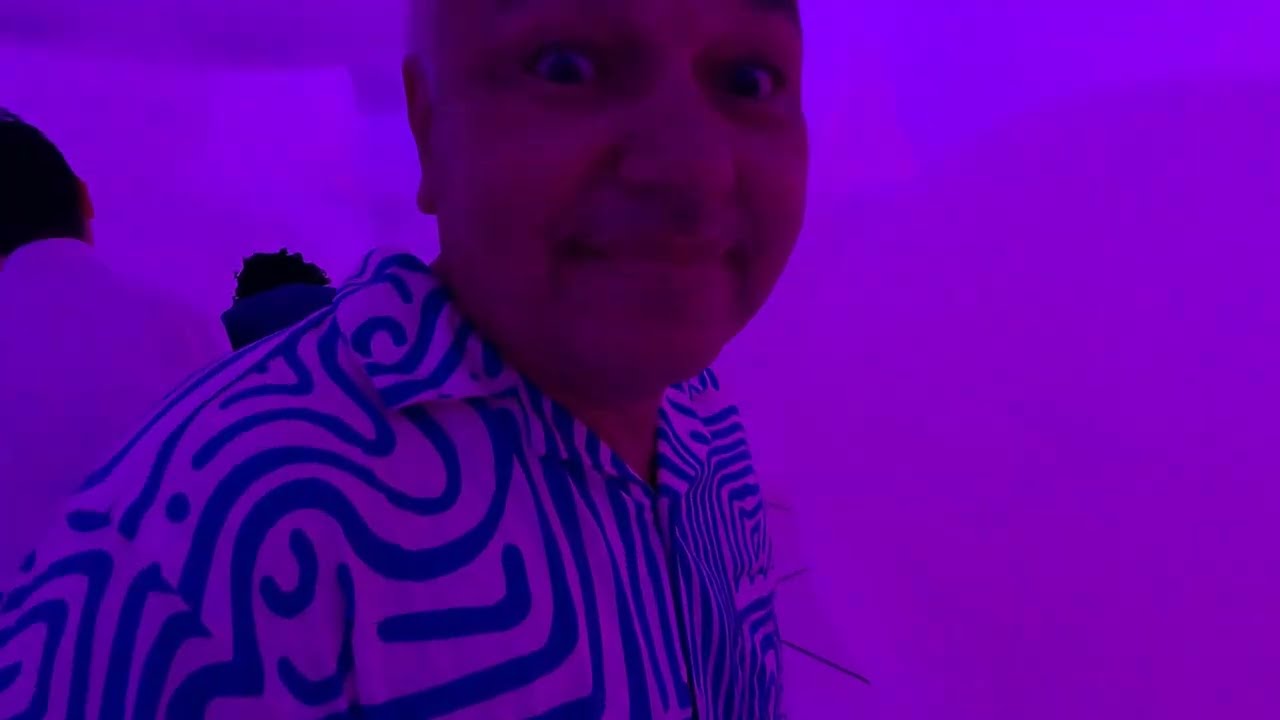The image is a horizontally aligned rectangular picture with a predominant purple background in various shades. It features a close-up of a man who appears to be looking directly into the camera. The top of his head is cropped off at the eyebrows, and we can see down to his chest. He has light brown skin and dark eyes, although their exact color is somewhat ambiguous. His mouth is closed, but his cheeks are pulled back, suggesting a slight smile or smirk. He appears to be bald or has white hair cut close to his head.

The man is wearing a white button-down collared shirt adorned with an intricate pattern of blue and possibly green or purple squiggly lines and geometric shapes. Behind him, on the left side of the image, are the indistinct backs of two other people. One person on the far left has short brown hair and is wearing a white shirt, while the second person to their right has spiky brown hair. The right side of the picture is devoid of any detail, emphasizing the purple background more extensively. Overall, the image gives a vivid sense of creativity and a filtered effect, capturing a moment that feels both intimate and expressive.